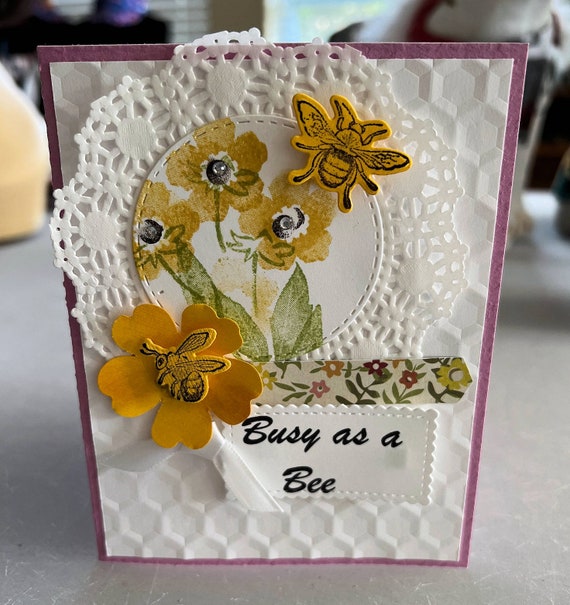This image showcases a meticulously handcrafted greeting card featuring several detailed elements. The background consists of purple construction paper overlaid with a textured white honeycomb-patterned paper. Adding to the layered design, a white paper doily is centrally pasted onto the honeycomb background. Adorning this doily is a circular, white, stitched leather disc, which serves as a canvas for three beautifully painted sunflowers embellished with black bead-like centers. A bee sticker or decal hovers near one of the flowers, adding a touch of whimsy. Additionally, there is a small cardboard cutout of a yellow flower with another bee decal attached to it, placed at the bottom of the doily. A dainty white bow graces the base of this artful composition, and finishing off the design is a white name tag with the cursive phrase "Busy as a Bee." This charming piece, potentially the front of a homemade greeting card, exudes a rustic and heartfelt charm, making it a unique, handmade treasure.